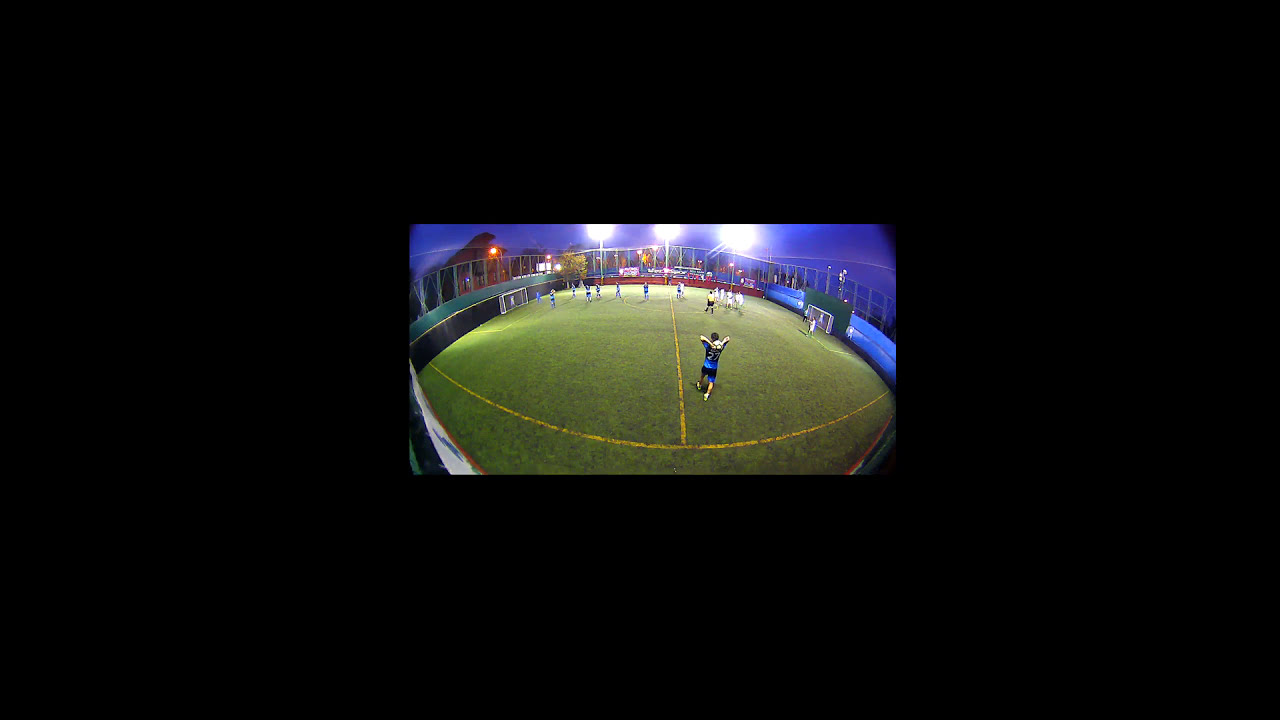In this image, a small central photograph is framed by a wide, black border that occupies about 80% of the overall space. The picture within the frame depicts an outdoor soccer field during the late evening, brightly illuminated by three spotlights positioned at the top center. The surface of the field is lush, green grass marked with vibrant yellow lines delineating the boundaries and center line of the game. Approximately twenty players populate the field, with some positioned along the center line. A prominent player is captured mid-throw in the center of the image, his back turned to the camera, with the ball poised behind his head. Goals flank either side of the field, marked in white, while the background features a variety of colors: blue fencing to the right, a reddish hue at the center back, and green with a black base on the left. The players are distinguishable by their uniforms, with the team on the right wearing white and the team on the left in blue. There is no text present anywhere in the image.